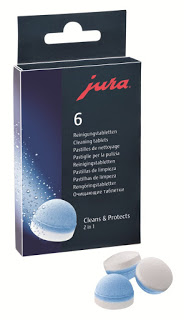In the image, there are two color drawings primarily featuring a product box prominently labeled "Jura" in red cursive text at the top right. The black box fades to blue on the left side and has a hanger tag at the top. Directly below the red "Jura" text is the number "6". The box's lower left corner shows a detailed, oblong cleaning tablet, which is predominantly sky blue on top and white on the bottom, with the blue portion covering approximately two-thirds of the tablet. Surrounding the tablet are illustrated bubbles, suggesting dissolution in water. The box also contains white text, detailing that the product consists of "cleansing tablets" and offers a "2 in 1" formula that "cleans and protects." Additionally, at the lower portion of the image, three more tablets are depicted. They share the blue and white coloration, with one tablet displayed face up and the other two oriented with their white sides showing.